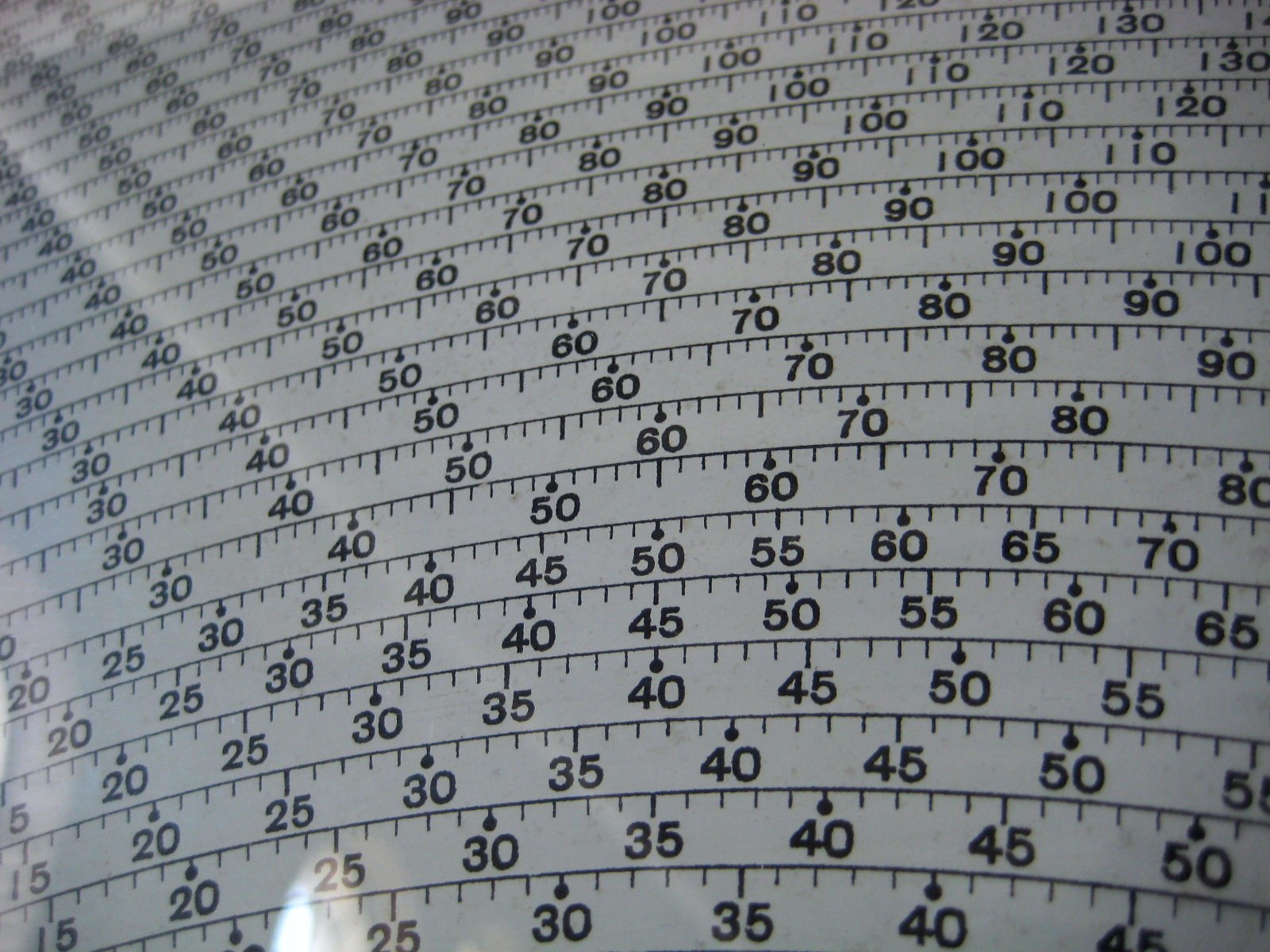The image showcases a collection of clothing tape measures typically used for measuring waist, thigh, and other body dimensions. Displayed on a sheet for the purpose of being cut into individual tape measures, the image features a series of white tape measures with black numerical markings. The bottom row of the sheet displays measurements in increments of 5, reading as 15, 20, 25, 30, 35, 40, 45, and 50. Moving upwards, the increments shift to every 10 units, showing 30, 40, 50, 60, 70, and 80. The lighting in the image creates a slight reflection, adding a touch of sheen to the overall scene.